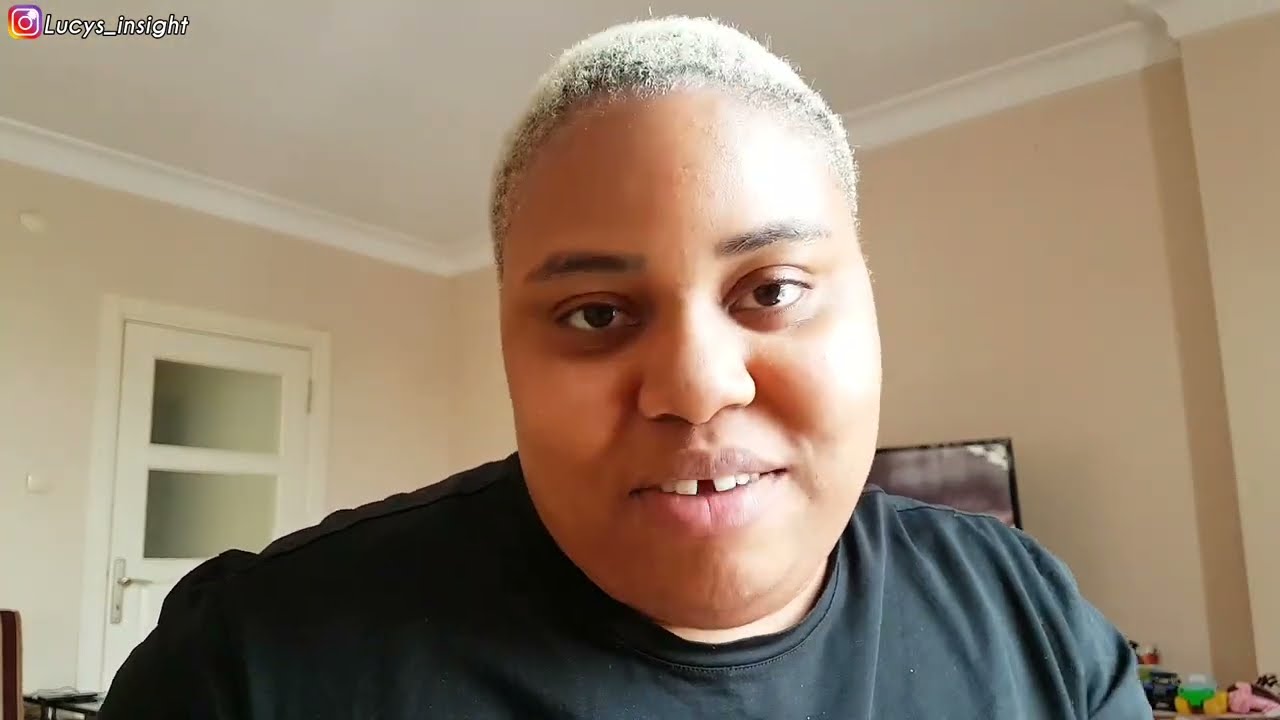This vibrant photograph from an Instagram account labeled "Lucy's Insight" prominently features Lucy, a young black woman with a distinct gap between her front teeth and striking short white hair. The landscape-oriented selfie captures Lucy in a black t-shirt, facing the camera with a warm half-smile that exudes friendliness. Dominating the composition, her expressive brown eyes draw the viewer's attention, while the background reveals a glimpse into her living space—a living room with beige walls, a white door featuring two paned windows, and a TV or computer monitor subtly blending into the decor. Scattered toys add a touch of everyday life to the serene setting. The Instagram logo in the top left corner, adorned with the handle "Lucy's_insight" in elegant white italic script, hints at a shared moment or a potential live stream, inviting followers to engage with Lucy’s latest insights.